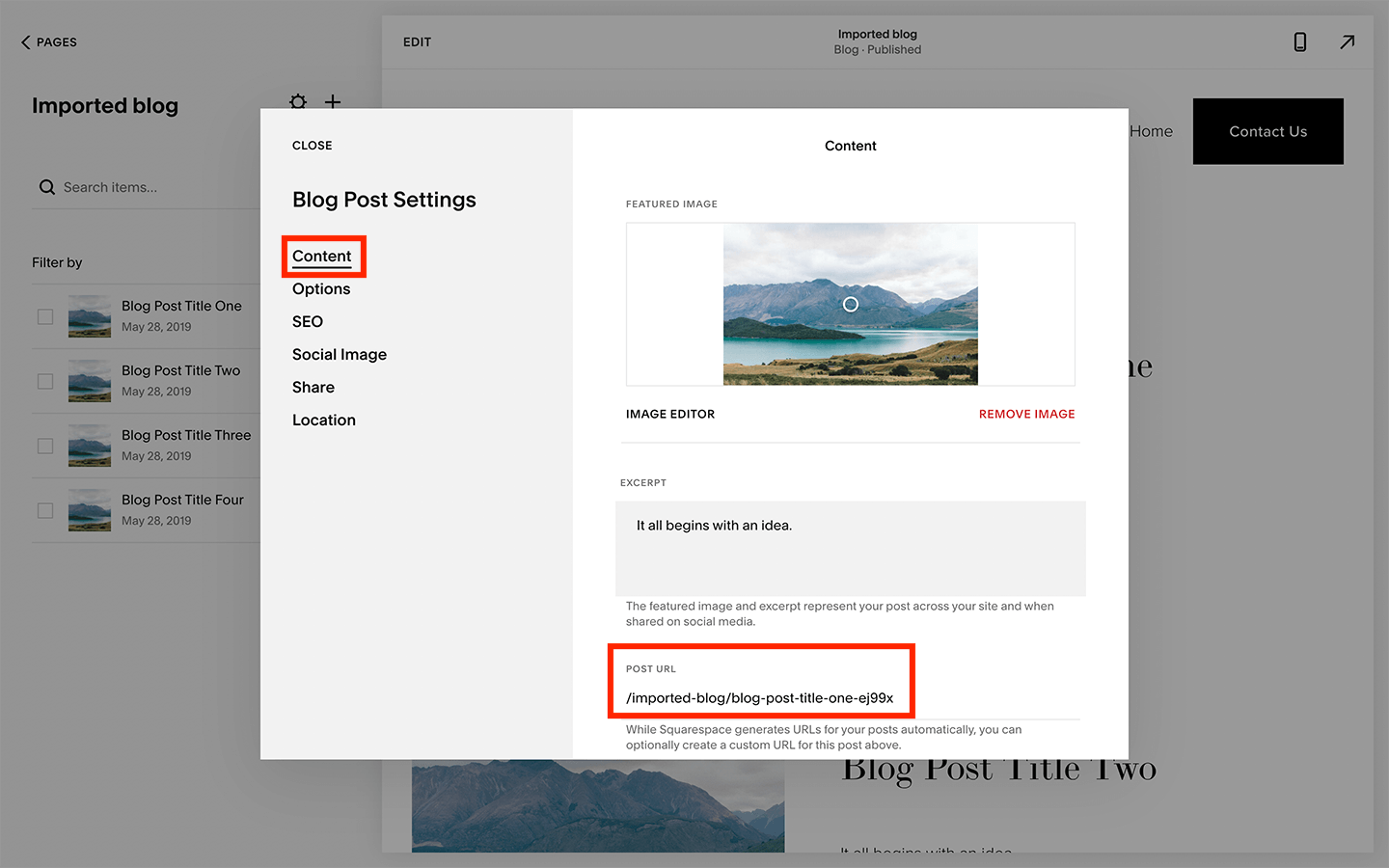### Detailed Descriptive Caption:

This screenshot displays a feature-rich blog post tool, likely integrated within a website builder like Squarespace. The focal point is a large rectangular sub-menu dedicated to blog post settings, positioned prominently in the center of the screen. The upper-left corner of this rectangle houses a close button for easy dismissal.

Below the close button, black text indicates various settings categories including content, search engine optimization (SEO), social image, share, and location options. A red rectangle underscores the currently selected 'content' menu. Another red rectangle highlights the 'post URL' section at the lower right-hand side of the screen. This section explains that while Squarespace generates URLs automatically, users can customize them.

To the left of the menu, the background reveals the main blog interface where users can search through existing blog posts. Four sample posts titled "Blog Post Title 1", "Blog Post Title 2", "Blog Post Title 3", and "Blog Post Title 4" are visible, confirming the tool's blogging capabilities.

At the top center of the content menu, there's a section for a featured image presented in landscape format, depicting a picturesque river flowing through a mountain valley. Below the image, there’s an editor feature for modifications. A 'Remove Image' option appears in red text on the right side. Additionally, there's an excerpt and title area with the heading "It all begins with an idea". The featured image and excerpt are crucial elements, as they represent the post across the site and on social media platforms.